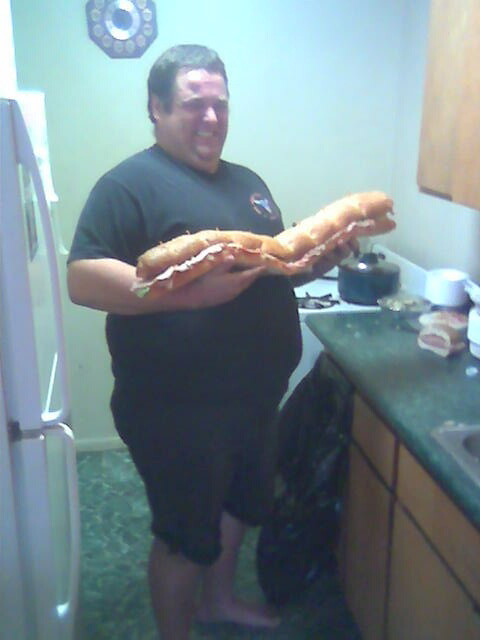A cheerful man stands barefoot in a small, galley kitchen, proudly holding an enormous sandwich that stretches nearly three feet, bending slightly in the middle under its own weight. He has a big smile on his face, short black hair, and is dressed in a black short sleeve t-shirt paired with dark shorts that reach just below his knees. The green-mottled floor complements the light blue back wall. To his left, a white refrigerator is partially visible, while to his right, a white stove with a black pot on top sits under light-colored wooden cabinets, partially in view. Directly in front of him is a green countertop housing a sink, with two brown drawers and cabinet doors below, and a plastic trash bag hanging off the edge. A few various items are scattered on the countertop, and a clock with hexagonal patterns and circular-number placements is mounted on the left wall. The overall coziness of the kitchen contrasts with the grandeur of the sandwich, making for a delightfully whimsical scene.